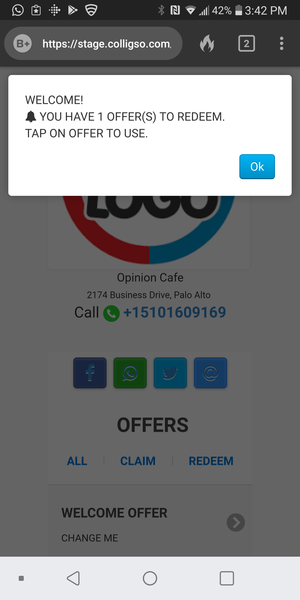**Detailed Descriptive Caption:**

This is a detailed screenshot of a smartphone screen taken at 3:42 PM, with the battery level at 42%. The device is connected to both cellular and Wi-Fi networks, showing 4 out of 5 bars for cellular signal strength and 3 out of 4 bars for Wi-Fi signal. Bluetooth is enabled. The primary application in use is WhatsApp, along with several other unidentified icons.

On the screen, a web browser is active displaying a web address, "http://stage.colleague". Next to the URL, there's a fire icon, a indication that two web pages are open, and a vertical three-dot menu icon for additional options.

A notification message below reads, "Welcome, you have one offer to redeem, tap on offer to use" with an "OK" button at the bottom of this notification box. In the background of this notification is a prominent logo featuring the word "Logo" surrounded by a red and blue circle.

Further down, the screen shows the text, "Opinion Cafe, 2174 Business Drive, Palo Alto" followed by a phone number formatted for WhatsApp, "Call WhatsApp 510-160-9196."

The combination of visible icons, notifications, and connections gives a comprehensive snapshot of the device's activities and status at the time of the screenshot.